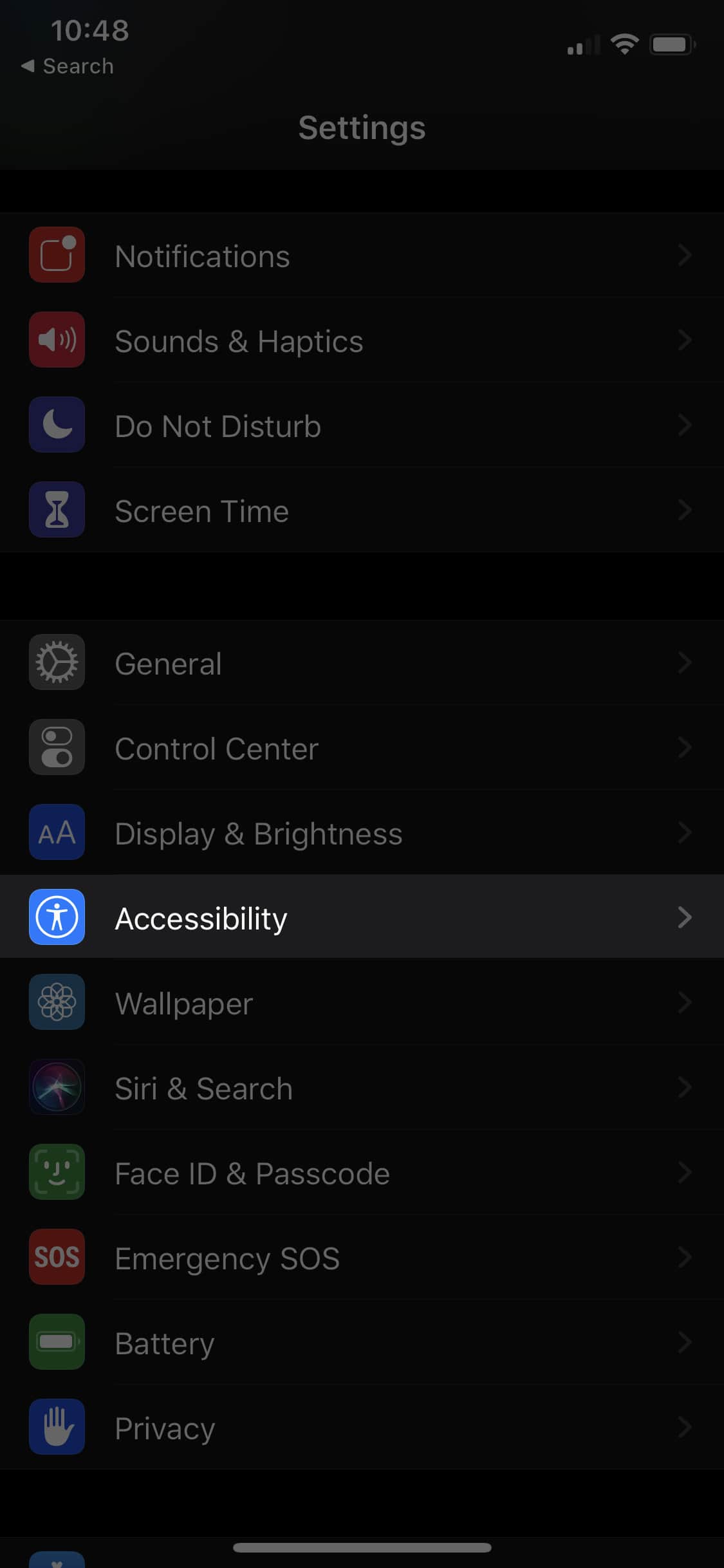The image is a screenshot from a smartphone displaying its settings page. The background is predominantly black with text in white and gray, providing a stark contrast for readability. At the top of the screen, the status bar is visible, indicating it is 10:48 AM. The phone has two out of four bars of cellular reception, an active Wi-Fi connection, and a nearly full battery, as shown by their respective icons in the upper right corner.

On the upper left, a back arrow and the word "Search" are displayed, suggesting navigational options for the user. The word "Settings" is prominently centered at the top of the page.

The settings are organized into two distinct groupings. The first grouping contains four categories: Notifications, Sounds & Haptics, Do Not Disturb, and Screen Time. The second grouping consists of ten categories: General, Control Center, Display & Brightness, Accessibility, Wallpaper, Siri & Search, Face ID & Passcode, Emergency SOS, Battery, and Privacy.

Among these settings, "Accessibility" is currently selected, distinguished by its bright white text, while the rest of the categories are in grayed-out text alongside their corresponding icons. The detailed depiction of the settings page and the precise icons alongside each category provide a clear and organized overview of the phone’s configuration options.